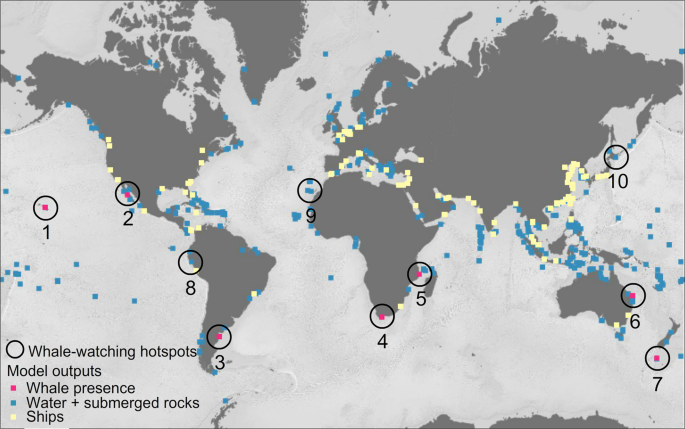The image displays a world map with light gray waters and dark gray landmasses, devoid of any detailed geographic features like cities or houses. The map features multiple black circles and colored dots—blue, yellow, and pink—strategically placed, mostly along coastlines. Situated in the bottom left corner is a key that deciphers these symbols: circles denote whale-watching hotspots, pink for whale presence, blue for submerged water and rocks, and yellow for ships. The map is labeled with numbers 1 through 10, highlighting specific regions: pink dots 1 and 2 are in the Pacific Ocean near North America; circles labeled 8 and 3 are around South America; dots 9 and 4 are off the west coast of Africa; circle 5 is placed east of Africa; dots 6 and 7 are east of Australia; and dot 10 is east of China and Japan.